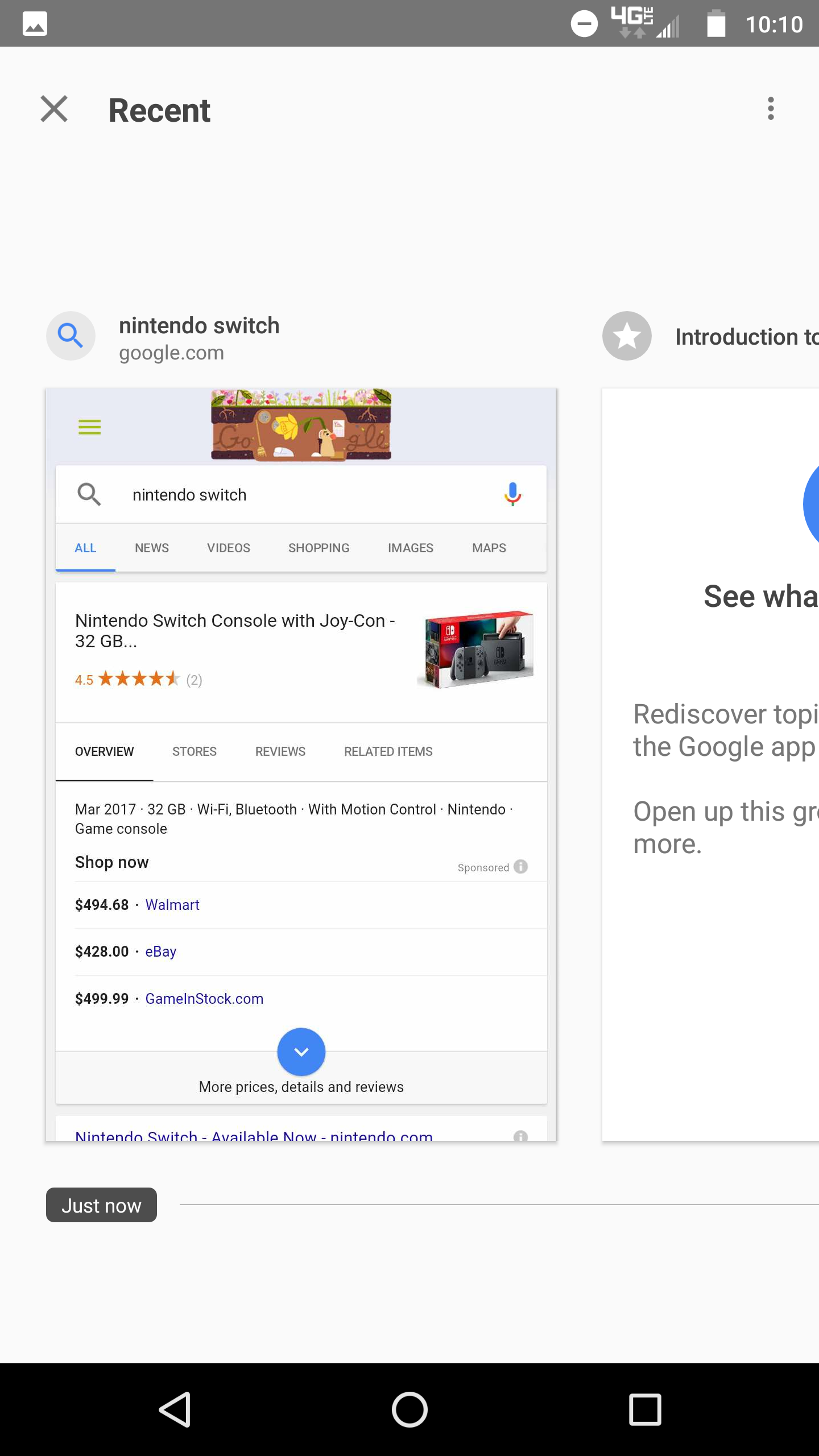The image is a screenshot captured from a mobile device, indicating the user is connected to a 4G LTE network with three signal bars and a battery life of approximately 90%. The time displayed at the top right of the screen is 10:10 AM.

The background of the screenshot is predominantly white with some black elements. At the very top, there's an 'X' button labeled 'recent.' The search query is visible in the search bar, beginning with a blue magnifying glass icon to the left of the text. The search bar reads "google.com," with a colorful Google banner positioned above it. The Google logo is set in a brown box adorned with flowers, adding a decorative element.

Below, the search results show information about the "Nintendo Switch Console with Joy-Con 32GB," which boasts a 4.5-star rating displayed in yellow. A red and white box featuring the Nintendo Switch console itself is prominently shown, including the black Joy-Con controllers.

Several tabs are visible: "Overview," "Stores," "Reviews," and "Related Items." The description mentions that the Nintendo Switch was released in March 2017, includes 32GB of storage, WiFi connectivity, and motion control features. There are multiple purchasing options listed: Walmart offers it for $494.68, eBay for $428, and GameInStock.com for $499.99. A "Shop now" prompt further encourages purchasing.